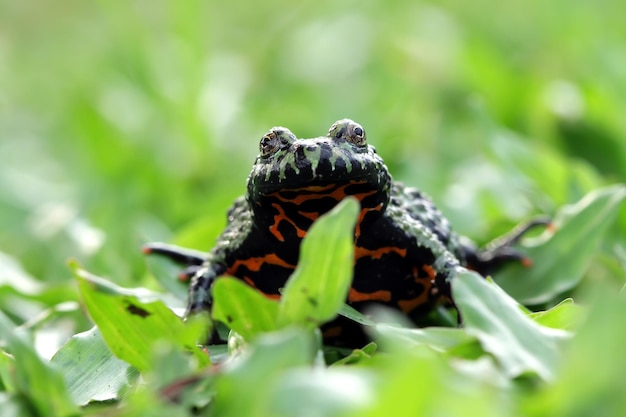This detailed color photograph captures a striking fire-bellied toad situated amidst a bed of green leaves. The toad, which appears large and prominent, is viewed head-on, showcasing its vivid and intricate coloration. Its skin on the dorsal side, or the top, exhibits a deep jet-black hue adorned with vibrant lime green web-like patterns, particularly on its face and back. Contrasting this, the ventral side, particularly beneath its throat and chest, displays irregularly shaped lines in a bright orangey-red. This color extends to its toes, adding to its vivid appearance. The background, though very blurred and green, reveals the leafy ground the toad rests upon, allowing the focus to remain sharply on the toad’s unique and colorful features.